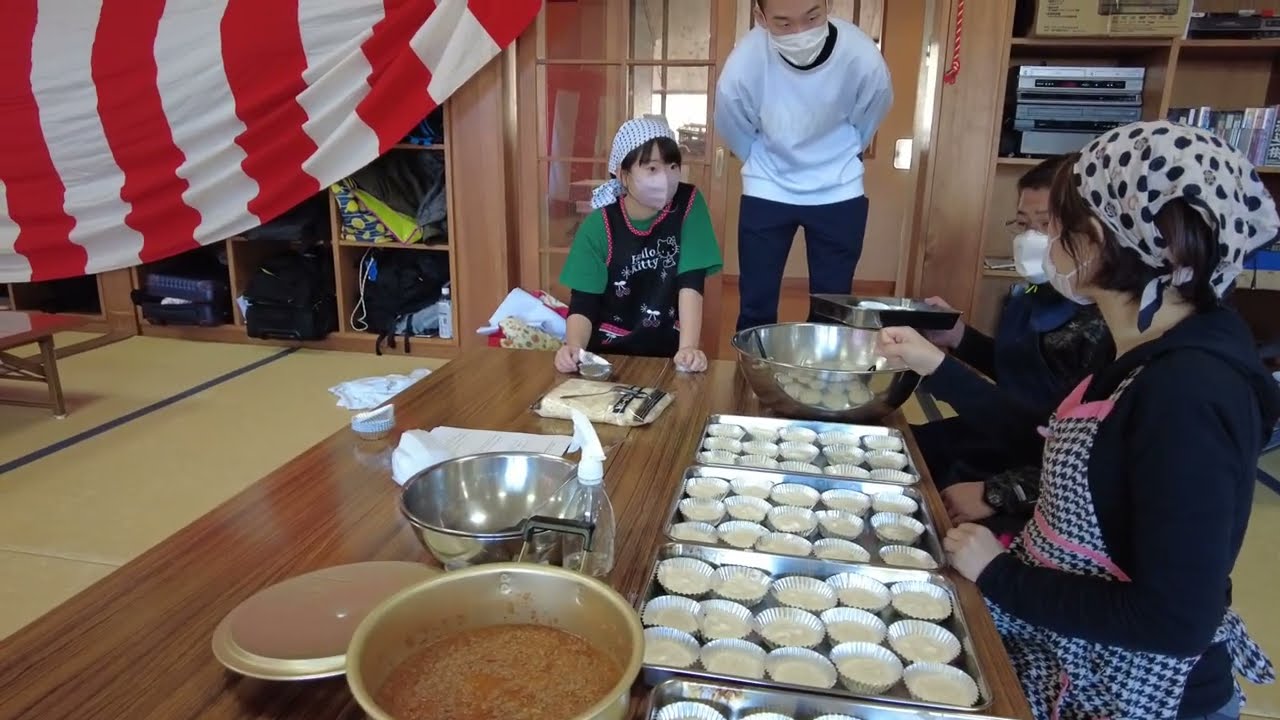In this detailed indoor scene, four individuals, likely Asian, are seen preparing a large quantity of food at a long dining table. They are in a space that resembles a classroom, evidenced by the shelves to the left filled with backpacks and a red and white banner that might be part of an American flag. The participants—two women and two men—are all wearing aprons, hair covers, and medical masks, suggesting a focus on hygiene, likely due to the food preparation. 

On the table, there are several aluminum trays with cupcake forms lined with paper cups. Some of these cups have a batter-like mixture, possibly chocolate, while others seem to contain a meat-based filling from a nearby pot with ground meat and sauce. This gives the impression that they might be making a traditional dish, perhaps tarts or meat pastries. The table is also equipped with several metal bowls, a water squirt bottle, and a pot, creating a busy, workshop-like atmosphere. 

One woman stands at the head of the table holding a large spoon, observing the others' work, while a man bends over, engaging with the participants. The scene encapsulates a communal cooking activity, rich with cultural undertones and meticulous preparation.